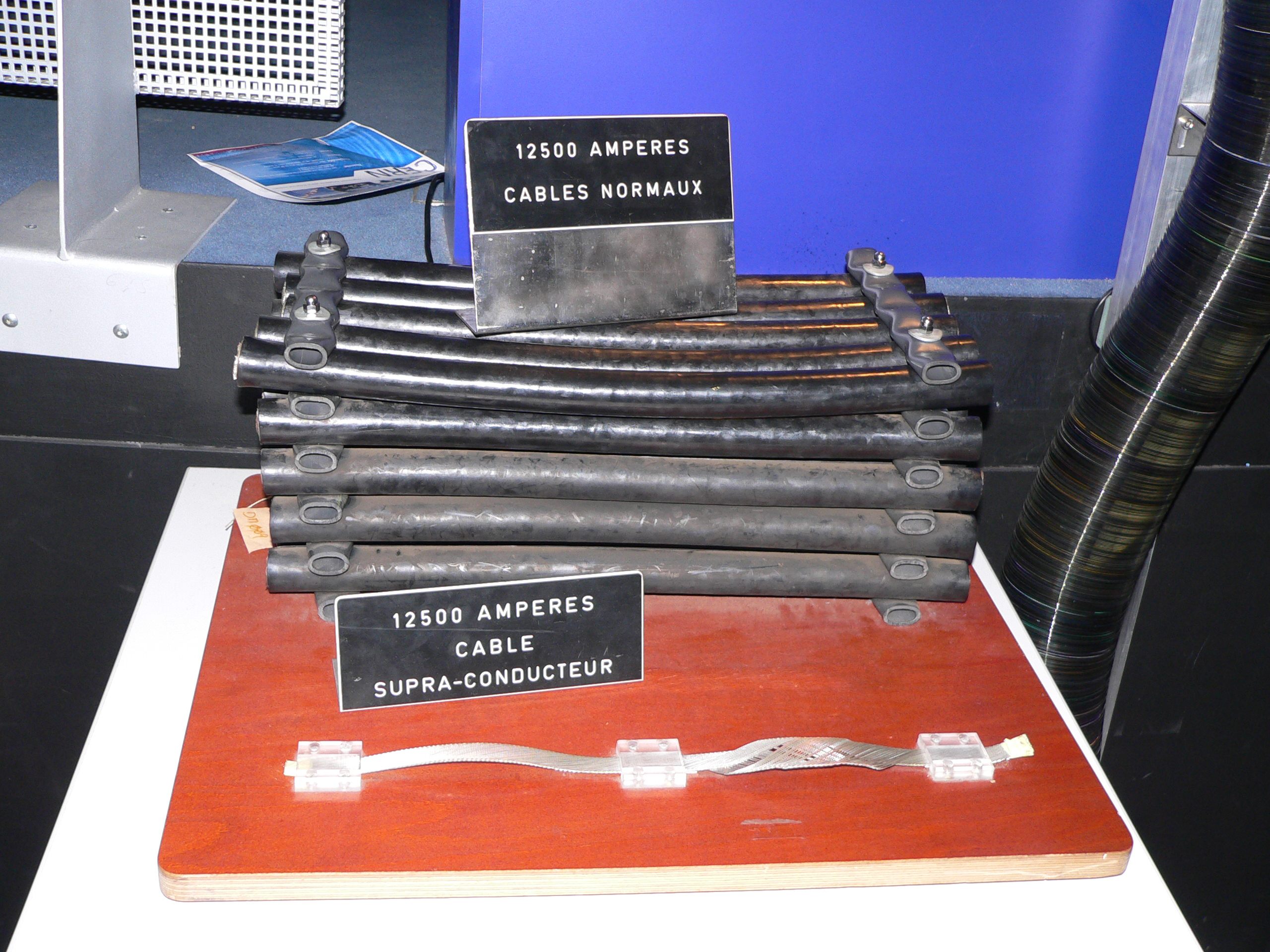The image depicts a display featuring a stack of thick, silvery cables. At the bottom, the cables exhibit a dull silver hue, which gradually transitions to a shiny silver toward the top. Attached to the cables is a metallic sign, overlaid with a black plastic label displaying white text: "12,500 Amperes." Beneath this, the sign reads "Cable Normaux," suggesting standard cables, written in French.

The cables and signage rest on a felt-like orange display board. The board's top section is orange, transitioning to another section at the bottom that features a flat-wired cable, similar to those commonly seen in computer setups. This section also bears a label stating "12,500 Amperes Cable Supraconductua," indicating these are superconducting cables, again noted in French.

The orange display board is placed on a white surface. To the side of the display, a round vent rises up, and in the background, a booklet can be seen resting on a counter. The image captures the details of the cables and signage, highlighting the contrast between the different types of cables and their respective current capacities.